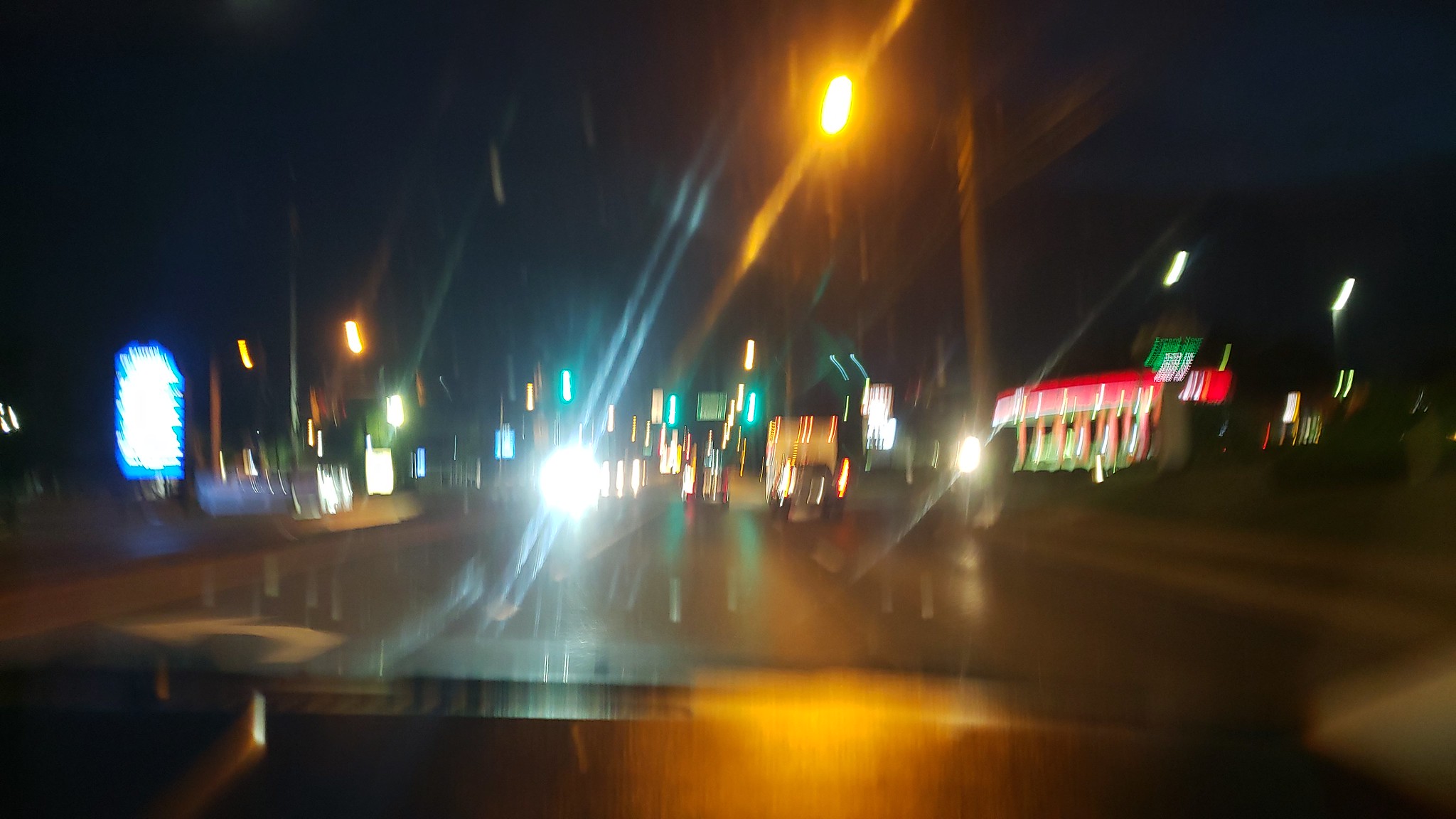The nighttime photograph, taken from the dashboard—perhaps even the passenger side—of a moving car, captures a blurry, light-streaked scene. Both the dark gray and black dashboard and the pitch-black sky indicate the hour. The car is driving on a dark gray road, with the blurry reflections of various lights adding to the scene's vibrancy. 

On the right, a business with red and green highlights and a billboard emits a blurry glow, its details obscured due to movement. Nearby, a gas station's stalls and roof are visible, casting more light into the scene. The dominant green traffic lights ahead and overhead yellowish streetlights add to the illuminated ambiance. Directly in front, cars can be seen with streaks of their lights extending through the image.

The left side showcases various traffic elements, including a white arrow on the road pointing left and a white and blue billboard. Amidst the blurred traffic lights and shapes, you can also identify a shopping area sign and green highway signs glowing in the distance. Street lights and a strong headlight from an approaching car create a white circle with light streaks, making the imagery even more dynamic and vibrant.